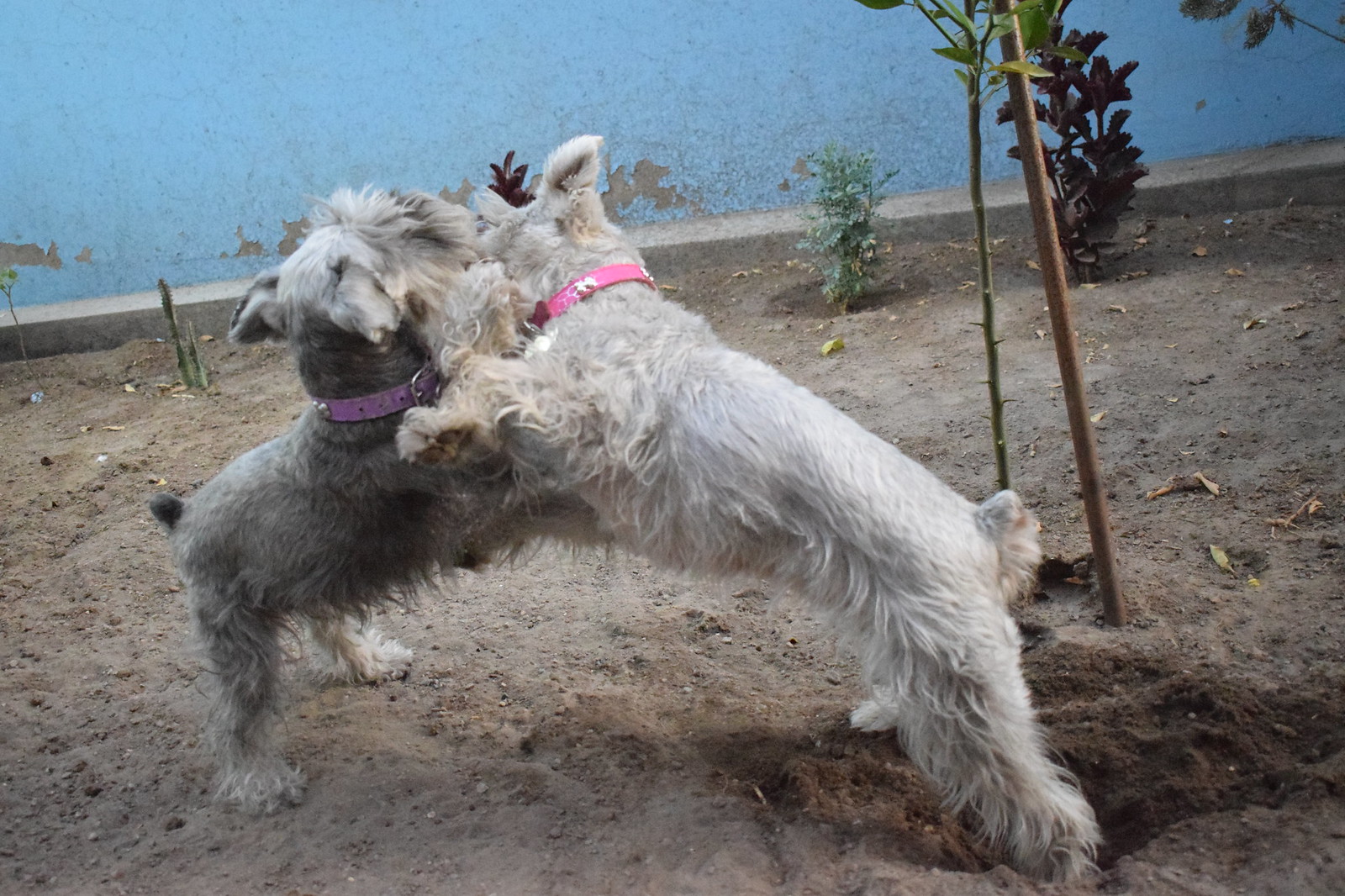In an outdoor setting that appears to be someone's backyard, two small, schnauzer-like dogs are captured mid-play, leaping towards each other on their hind legs. Both dogs have fluffy faces and docked tails, and they stand on a dirt ground amidst newly planted shrubs and a staked young tree. The backdrop features a light blue painted wall with patches of worn paint revealing the gray stone beneath. The dog on the left has a dark gray coat with lighter face and ears, wearing a purple collar, while the dog on the right sports a dirty white coat with a pink collar. They are engaged in a playful tussle, their front legs on each other and faces pressed closely together, radiating the energy of their joyous interaction.